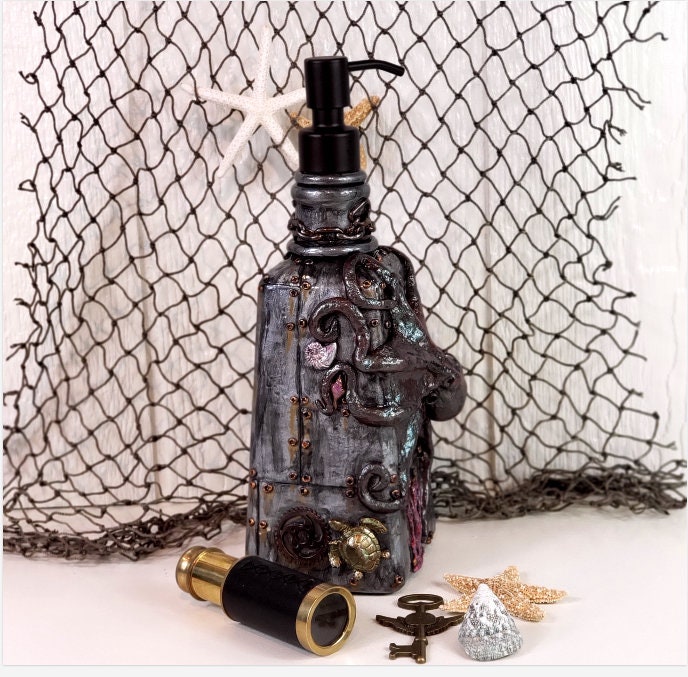In an indoor setting flooded with bright light, an unusual soap dispenser takes center stage. Designed in a boat-like, rectangular shape, the dispenser features a metallic gray body adorned with intricate engravings of sea creatures, including a gold turtle and a decayed-looking octopus. The top is black, designed for pressing to dispense soap, adding to its vintage, somewhat distressed aesthetic. Surrounding the dispenser, you'll find a collection of marine-themed items: a miniature telescope in gold and black, an antique-looking key, a starfish seashell, a pointed light-colored seashell, and some pink, green, and white pearlized shells. In the backdrop, a worn fishing net hangs against the wall, showcasing a white starfish and a brown starfish, contributing to the maritime decor. The overall scene evokes an underwater treasure trove, albeit with a somewhat deteriorated charm.